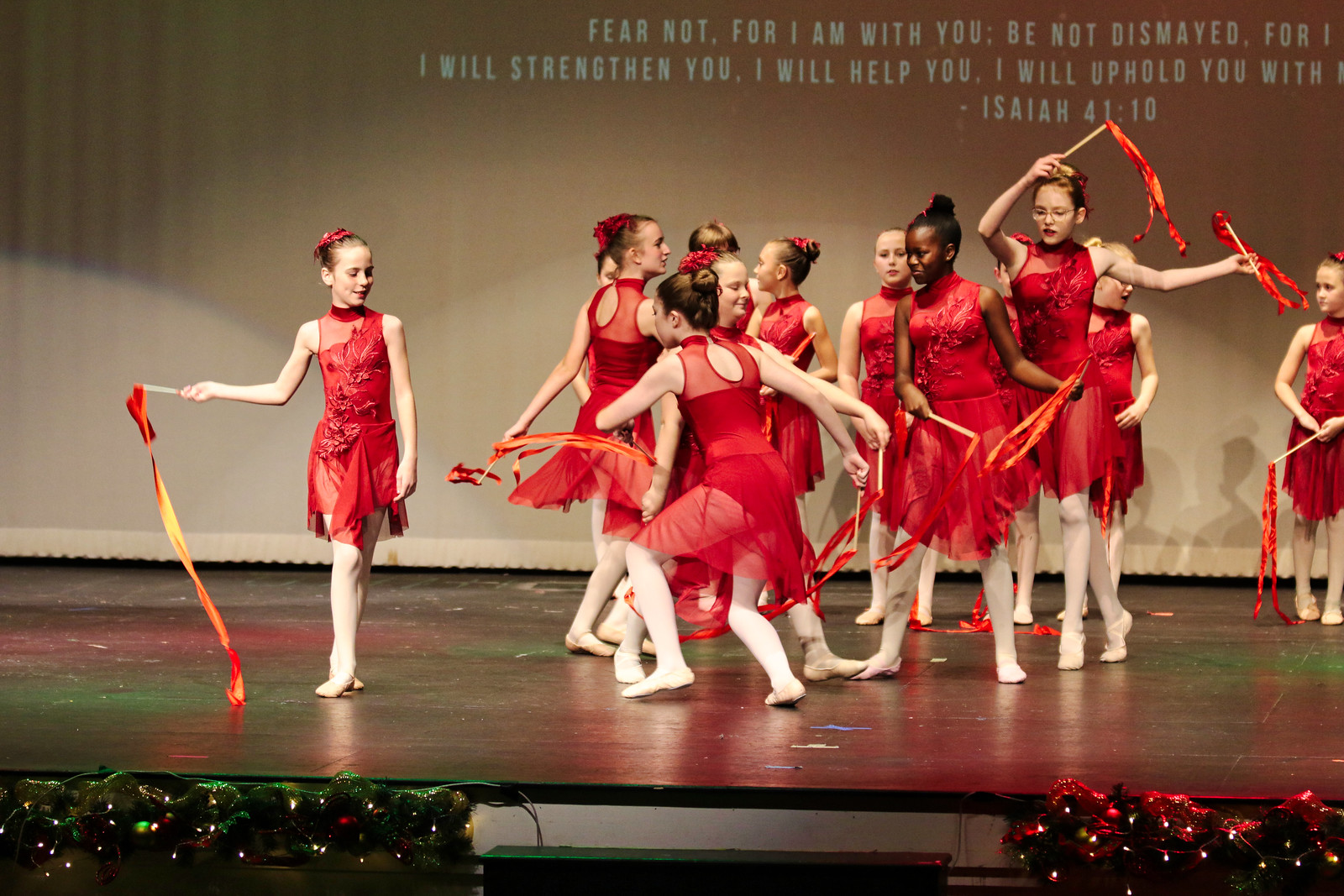The image depicts a group of young school-age girls performing a dance on a stage. They are dressed in red ballerina costumes with white tights, their hair up in tight buns adorned with red hairpieces. Each girl holds batons with red and yellow streamers, adding vibrant color to their movements. The central group forms a circle, with individual dancers positioned separately on the left and right sides. One girl is running around the group’s periphery. The black stage floor features markers and is illuminated by red and green stage lights, reflecting the festive theme. Along the front edge of the stage, Christmas-themed garlands are adorned with acrylic lights—green to the left and red to the right. Projected on the curtains behind the dancers is a Bible verse in white text: "Fear not, for I am with you; be not dismayed, for I will strengthen you. I will help you; I will uphold you with my righteous right hand. Isaiah 41:10," suggesting the performance might be part of a Christmas recital. The dancers appear to be preparing for their performance, not yet in synchronized motion, but rather setting up and finding their positions.